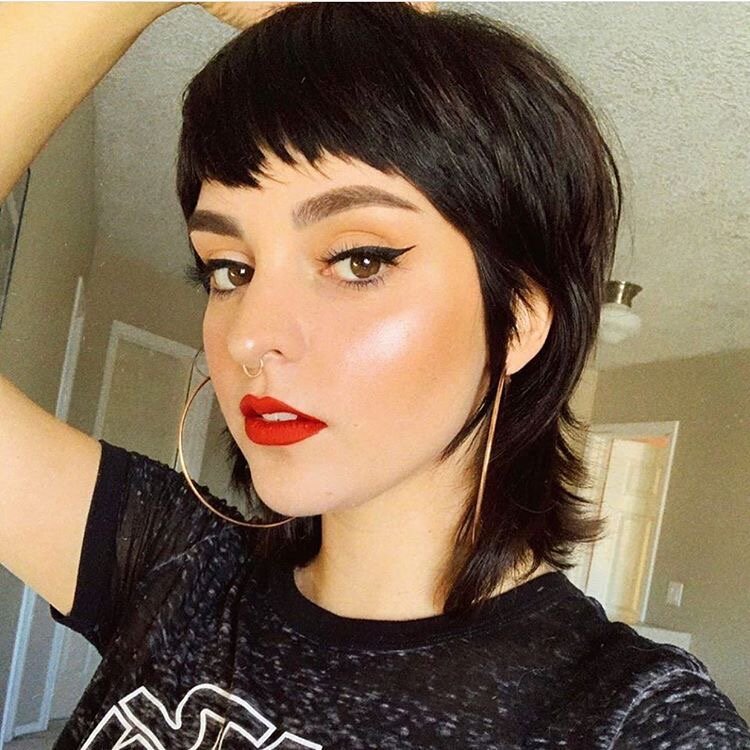The image showcases a young woman with short, shoulder-length, shag-style brown hair and bangs, posing for a selfie in a room with off-white walls and white, gold-based ceiling light fixtures. She sports bright red lipstick and black eyeliner, enhancing her glowing complexion. Her look is further accentuated by large hoop earrings and a gold nose ring. She is wearing a short-sleeved black t-shirt with white specks, possibly a Star Wars theme, adding a touch of shine or glitter. In the selfie, she has her right arm bent, with her hand resting behind her head, capturing a classic goth girl aesthetic. The vertical image has a realistic yet slightly filtered look.